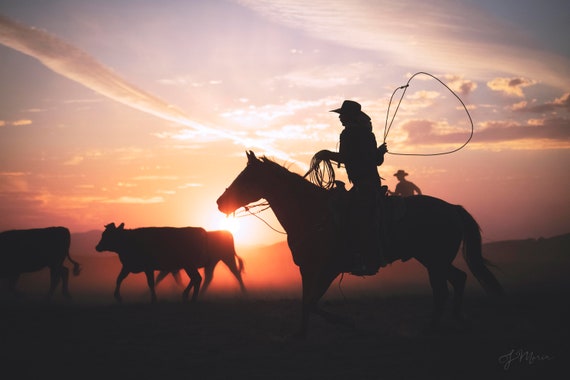The photograph captures a dramatic scene of two cattle wrestlers, silhouetted against the vivid backdrop of a sunset or sunrise. The primary focus is on the foreground wrestler, who is mounted on a horse and gripping its reins with one hand, alongside an extra loop of thin rope. In the other hand, the wrestler is skillfully spinning a lasso. Both wrestlers are dressed identically in long-sleeve coats and cowboy hats, with the second wrestler partially obscured by the first one's horse. The scene is cast in striking contrast due to the backlighting, turning the figures into black shadows. Three cows in front of the horse add to the composition, also appearing as dark outlines. The sky enhances the atmosphere with shades of dark purple, blue, and orange streaked across, further illuminated by the gold light of the sun sitting low on the horizon.